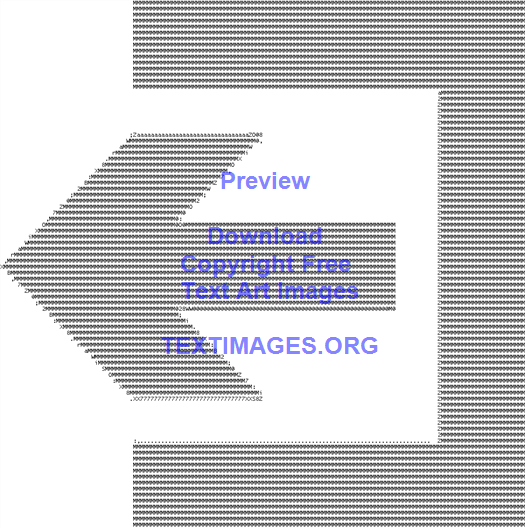The image depicts a piece of ASCII art resembling a backwards "C" or an incomplete rectangle with an open left side, evocative of a three-sided box encircling an arrow. This arrow is pointing to the left and is composed of numerous tiny characters, such as dots, numbers, or letters, though the exact details are blurred. The shapes are rendered in black on a white background. Centered within the image, in colored text, are the words: "PREVIEW" followed by "Download copyright free text art images" and "textimages.org." The artwork appears to be an advertisement promoting text art images available on the website textimages.org.